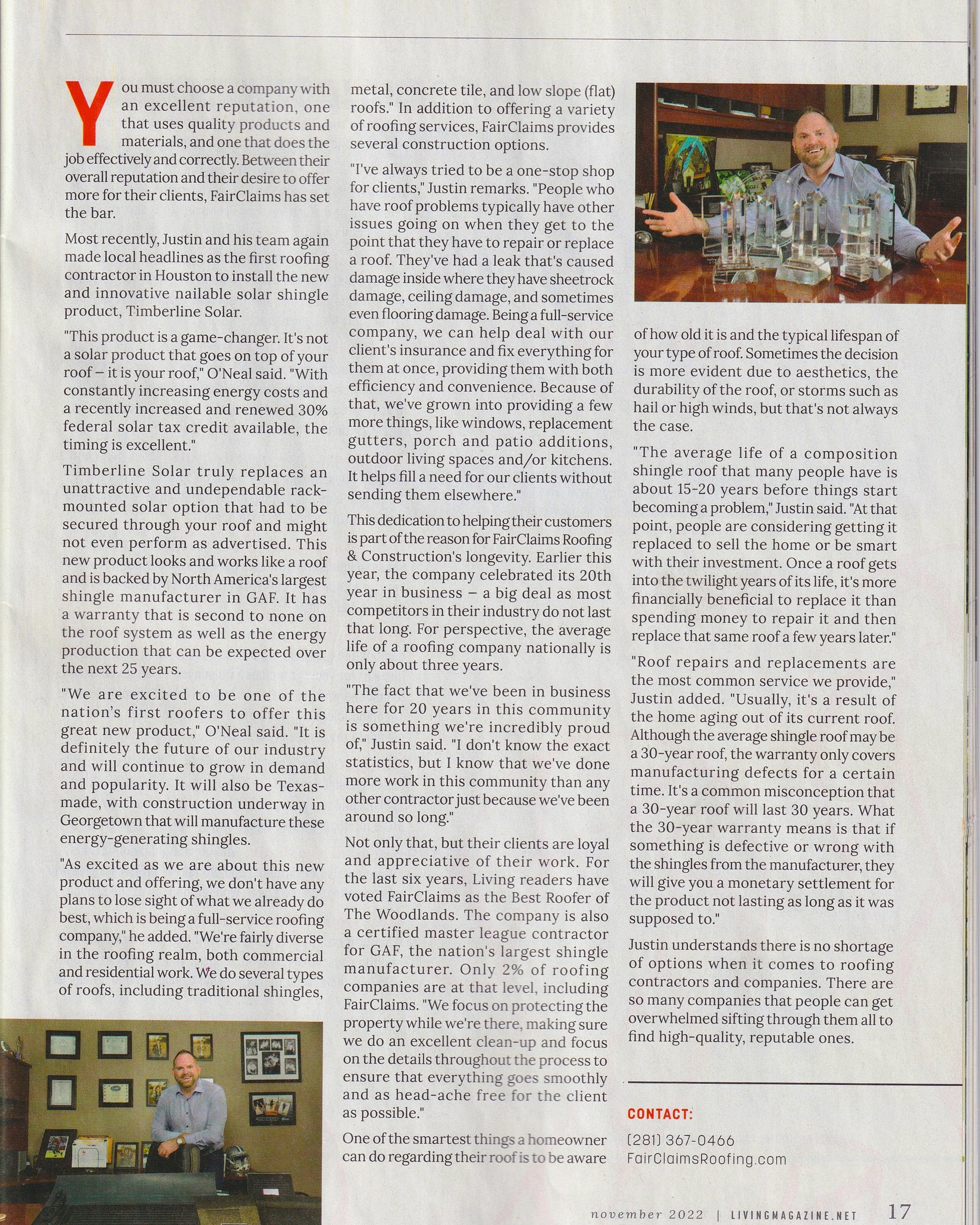The caption for the image could be:

"In this photo, we see Justin, a prominent figure featured in a recently torn-out magazine article, sitting proudly in front of an impeccably organized wooden desk. The background reveals an impressive array of plaques, awards, and accolades adorning the wooden shelves and cubby holes, showcasing his many achievements. Dressed in a comfortable long-sleeve shirt, Justin's open arms and welcoming gesture invite us to appreciate the multitude of honors he has received. 

The accompanying article highlights the exceptional reputation of his company, Fair Claims, renowned for its high-quality products and excellent service. Specifically, the article discusses Timberline Solar, a revolutionary product that integrates solar technology directly into the roofing material, eliminating the need for traditional solar panels. 

Justin's commitment to quality and client satisfaction has set a benchmark in the industry. He acknowledges the overwhelming number of roofing contractors available but emphasizes the importance of choosing reputable companies. Another image within the article shows Justin in a different setting, yet again surrounded by a testament to his success and dedication to his craft."